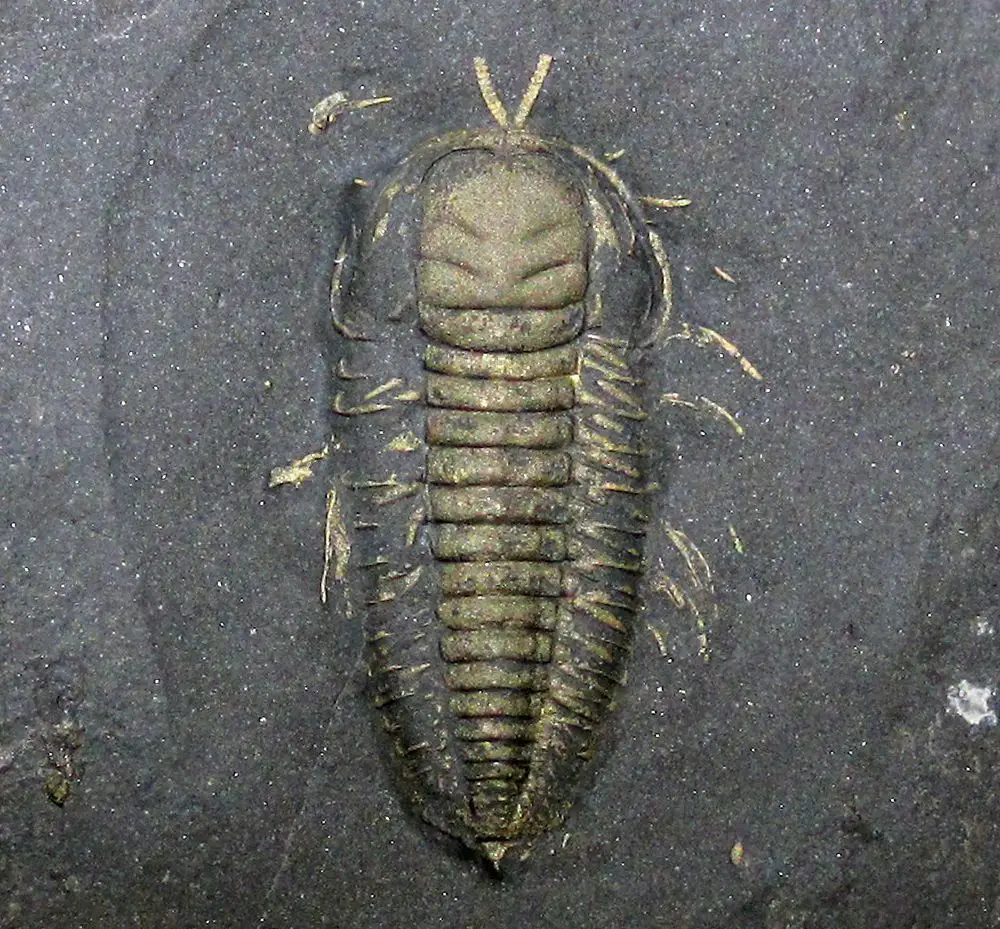The image showcases a photorealistic depiction or photograph of what appears to be a golden-brown ancient isopod-like creature, fossilized and inset into a dark gray rock. Dominating the center of the image, the creature spans nearly the entire vertical length, from top to bottom. Its large head area, situated near the top, features two prominent protruding mouthpieces. The creature’s segmented body and individual back spines are clearly visible as they extend towards its posterior. On the right side, several appendages are partially buried within the dark rock. The creature resembles a prehistoric insect, akin to a cockroach, with its body framed by what seems like a shell and legs that are partially revealed. The fossil is distinctly lighter in color compared to the dark, almost black, surrounding rock, creating a strong contrast. This image, devoid of any other objects, animals, people, numbers, vehicles, or text, captures the intricate details of the fossil, accentuated by the bright and clear natural daylight, suggesting an outdoor setting.